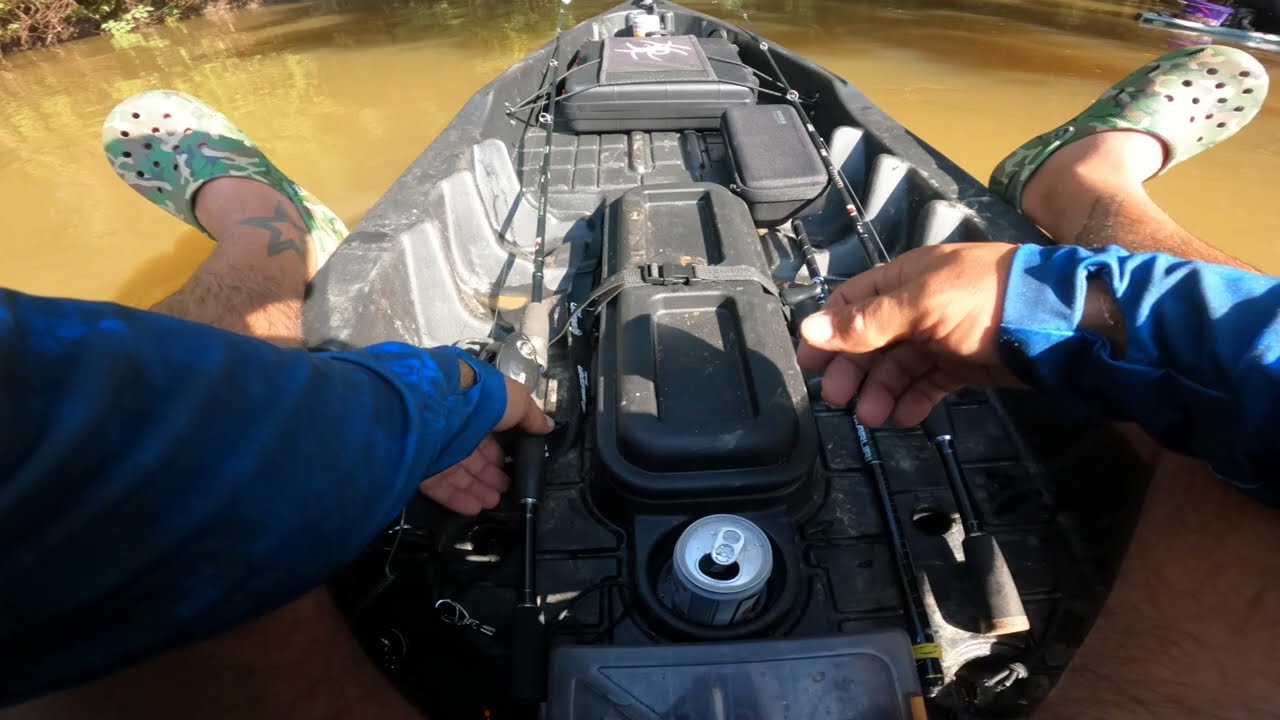The image depicts a point of view shot from a man seated in a kayak on a caramel-brown river or creek during the daytime. He is wearing a blue long-sleeve shirt, and his legs, adorned with camouflage-patterned Crocs and a star tattoo on the left foot, rest inside the gray interior of the kayak. His hands and arms, clad in the same blue shirt, are visible. In between his legs is an aluminum soda can nestled in a cup holder. The kayak contains various items, including a black container with a gray strap, a gray briefcase, and fishing gear such as rods and multiple strapped-down cases. The water is a light caramel brown, and small landing and brush are visible in the upper corners of the photo.